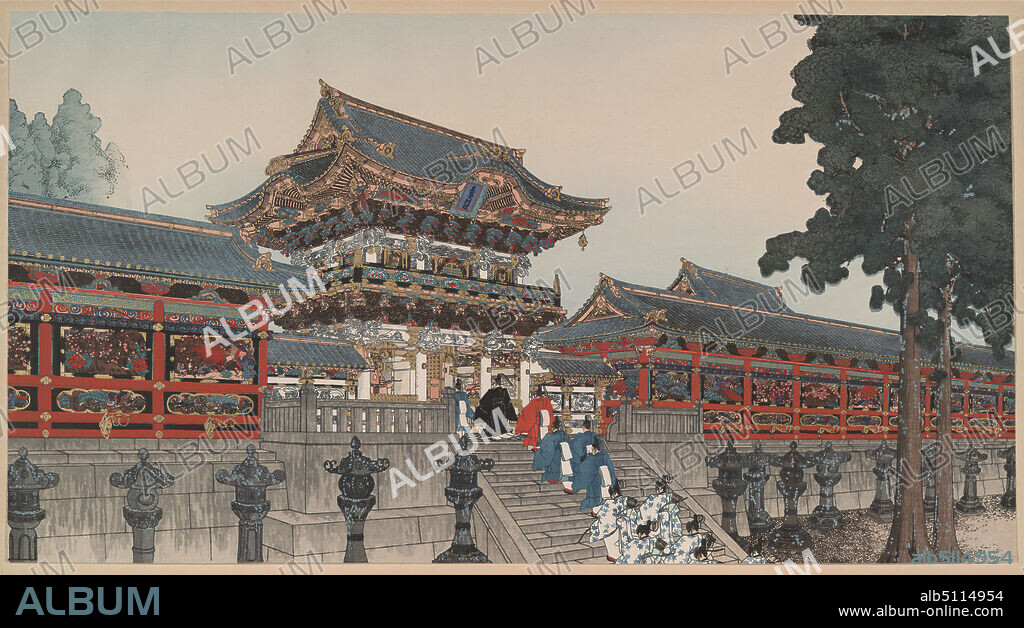The poster features an intricate watercolor painting of a ceremonial Asian-style building, likely from China or Japan, marked by its prominent central concrete staircase. Traditional Asian architecture dominates the scene, with a large stone wall at the bottom and platform stairs adorned with red decorations. Pillars, possibly for candle placements, flank the steps, adding to the ceremonial feel. The sky is a blend of light brownish-gray tones, featuring the faint outline of a tree on the upper left and more trees with green foliage on the right. The stairs are crowded with figures in traditional attire. Men, positioned at the front, wear a variety of colors, including red, black, blue, and green, while women at the back are dressed in white and blue flowery kimonos.

The image is overlaid with the word "album" repetitively, varying in dark, gray, and white fonts that serve as a watermark. A black horizontal strip at the bottom of the poster contains the text "ALBUM" on the left and "ALB 511-4954" along with the URL "www.album-online.com" on the right.